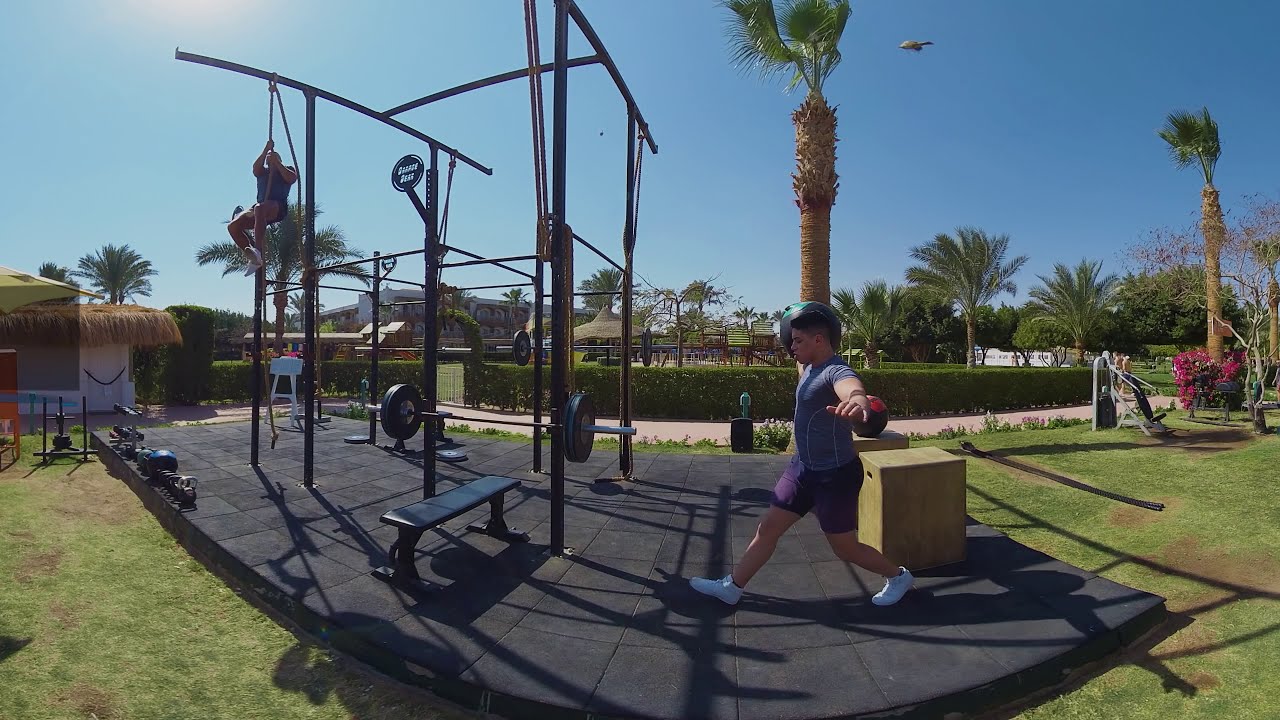In a vibrant outdoor gym set up on a lush, green grass field, a man in a tight spandex t-shirt, purple shorts, and white sneakers is balancing a large workout ball in his right hand. He stands on a black platform scattered with free weights and various exercise contraptions. To his left, there is a bench press machine, and further down another man can be seen climbing a rope attached to the apparatus, which is mounted on the six-inch-high platform. The sunny day highlights the bright blue sky, dotted with a helicopter flying by. Surrounding the gym are tropical plants, including palm trees and bushes, enhancing the park-like, healthy atmosphere.